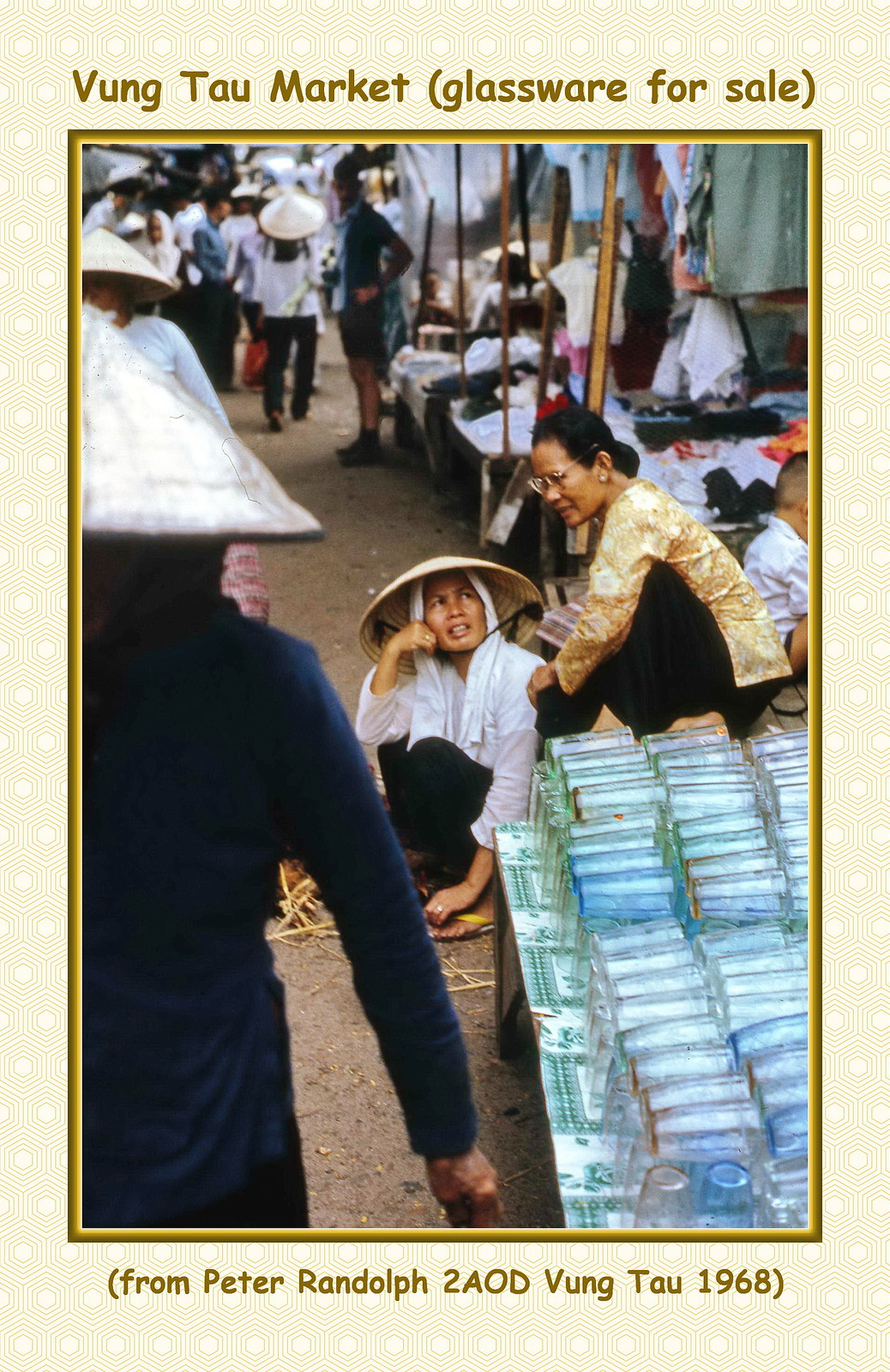This image is a photograph framed within a vertical rectangular card with a light tan border, thicker at the top and bottom, outlined in gold. At the top of the border in gold lettering are the words "Vung Tau Market" with "Glassware for Sale" in parentheses. The bottom of the border contains the caption, also in parentheses, "from Peter Randolph to AOD Vung Tau 1968."

The central focus of the photo is two vendor women at a bustling street market in Vietnam. The woman on the left is seated on the ground, wearing a traditional rice hat with white straps, a white top, and black pants. Her right hand is raised near her face, while her left hand rests on the ground. To her right, another woman is seated slightly higher, possibly on a bench or platform. She wears a yellow shirt, black pants, has black hair, and is wearing glasses. In the foreground on the bottom right, there are pallets with clear drinking glasses for sale. On the left, a person in a blue shirt with a rounded hat appears with their back turned to the camera, partially cut off at the waist, with their right arm extended downward.

Behind the women, there is a busy background featuring more market activity. Several people stand along a path, including one individual on a bicycle, hinting at the lively atmosphere of the market. To the right side in the distance, various objects and possibly a structure can be seen, further depicting the vibrant and chaotic essence of Vung Tau Market in 1968.